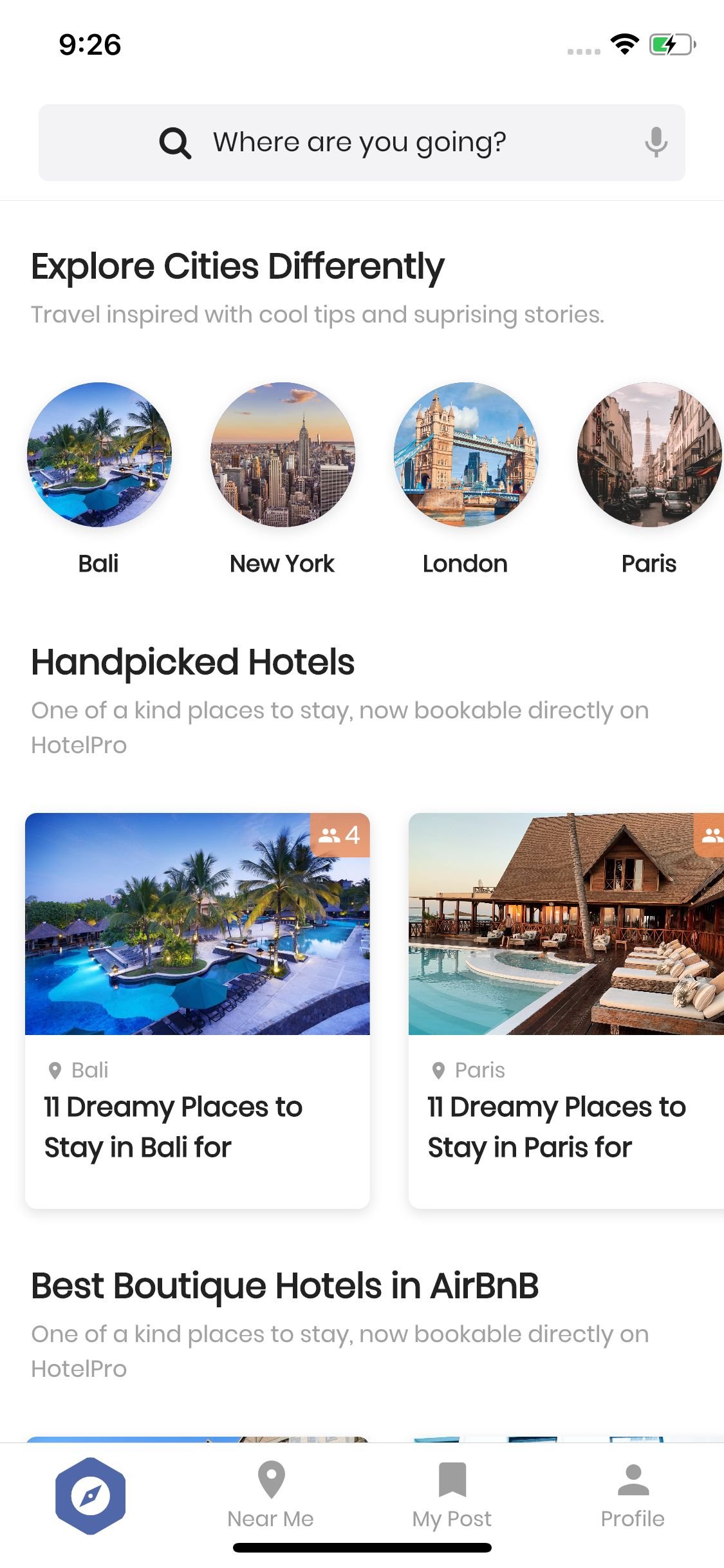The image displayed on the smartphone screen shows a user's travel application interface.

**Top Section:**
- **Time:** The time is displayed in black text as "9:26" in the top left corner.
- **Battery Status:** On the far right, a half-full green battery icon with a black thunderbolt is visible.

**Search Bar:**
- **Appearance:** A light gray search bar spans across the screen beneath the top section.
- **Icons/Text:** A magnifying glass icon is on the left, and a microphone icon is on the right. The text inside the search bar reads, "Where are you going?"

**Main Content:**
- **Header Text:** On a white background, bold black text states, "Explore cities differently."
- **Subtext:** Smaller gray text underneath reads, "Travel inspired with cool tips and surprising stories."

**Featured Locations:**
- **Destinations:** Four circles, each containing an image of a destination, are lined up from left to right.
  - **Bali:** An image of a tropical destination.
  - **New York:** An image likely showing an iconic New York landmark.
  - **London:** An image featuring a recognizable part of London.
  - **Paris:** An image of a Parisian scene.

**Handpicked Hotels Section:**
- **Header Text:** Black text stating, "Handpicked hotels."
- **Subtext:** Smaller gray text beneath reads, "One-of-a-kind places to stay, now bookable directly on Hotel Pro."

**Hotel Highlights:**
- **Bali Feature:**
  - **Image:** A photo of an infinity pool at a resort.
  - **Text:** Black text under the image reads, "11 dreamy places to stay in Bali."

- **Paris Feature:**
  - **Image:** A photo of an outdoor pool with deck chairs, likely at a lodge-style resort.
  - **Text:** Black text under the image reads, "11 dreamy places to stay in Paris."

This detailed caption provides a comprehensive description of the travel app interface displayed on the smartphone screen.